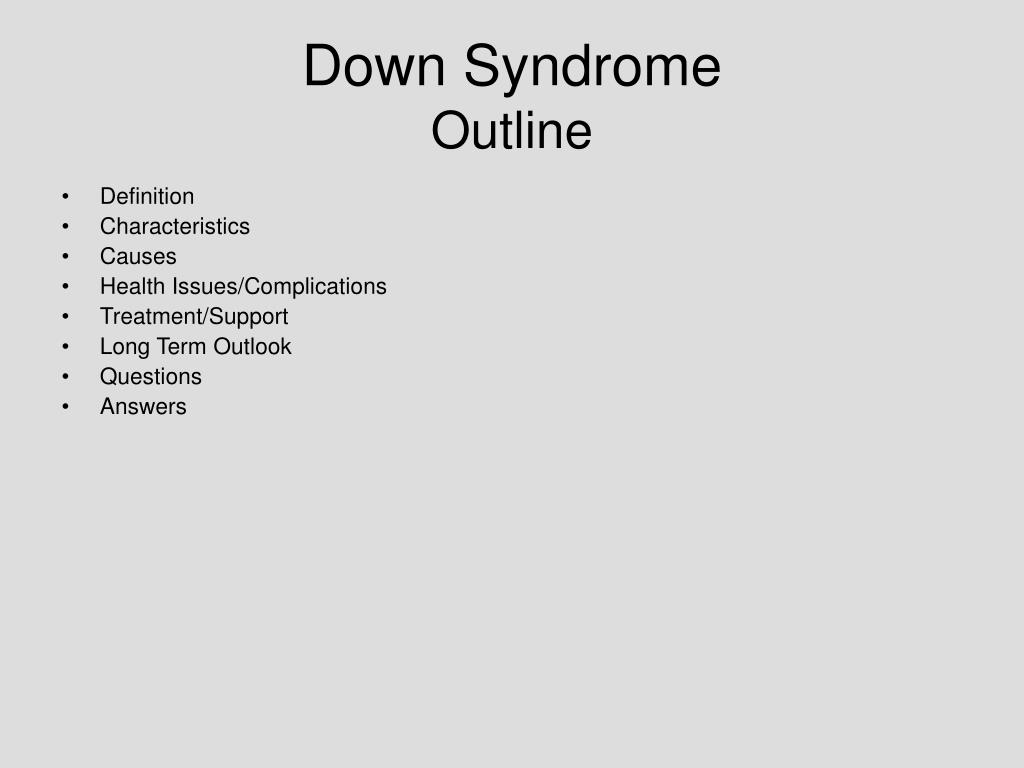This image showcases a detailed, text-heavy slide from a presentation with a gray background. The slide is structured with several key sections, each marked by a bullet point, outlining: Definition, Characteristics, Causes, Health Issues, Complications, Treatment, Support, Long-Term Outlook. Each section consists of 8 distinct bullet points that further elaborate on the topics. The layout includes a clear heading and individual bullet points to present extensive information effectively, resembling a classic slideshow format aimed at providing a comprehensive overview of a certain subject.